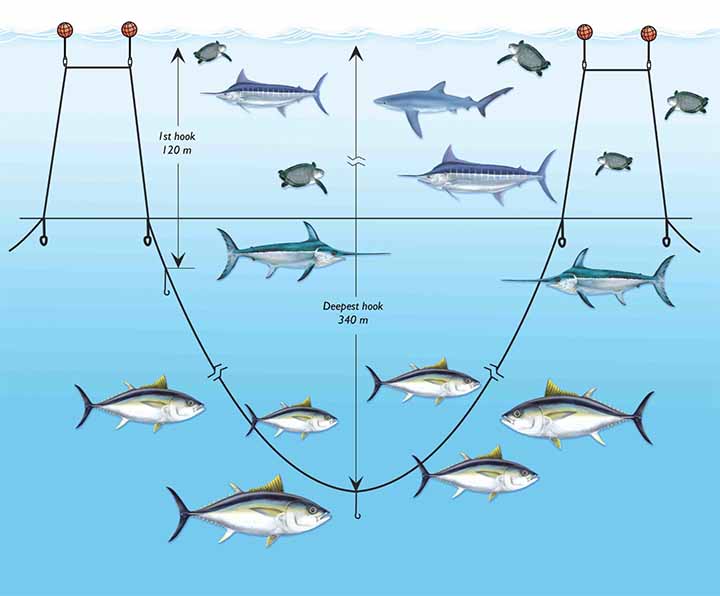The infographic illustrates the optimal depths for setting hooks to catch various types of fish in the ocean. The image, characterized by a light blue color reminiscent of water, depicts three different depth zones populated by distinct marine life. The surface layer around 120 meters deep features sea turtles, an assortment of smaller fish, a tuna, a shark, and a few swordfish. Moving deeper to the middle zone at around 240 meters, two swordfish are prominently displayed. At the greatest depth of 340 meters, larger fish with silverish bodies and black stripes dominate, indicating their preference for these deeper waters. The graphic also includes a depiction of ripply waves at the top, reinforcing the oceanic setting and suggesting that these fishing tips are suited for both casual pier fishers and those on fishing vessels. Various hooks and their corresponding depths are shown to guide users on the best fishing strategies. Additionally, there are nets depicted, adding to the comprehensive fishing instructions provided by the infographic.